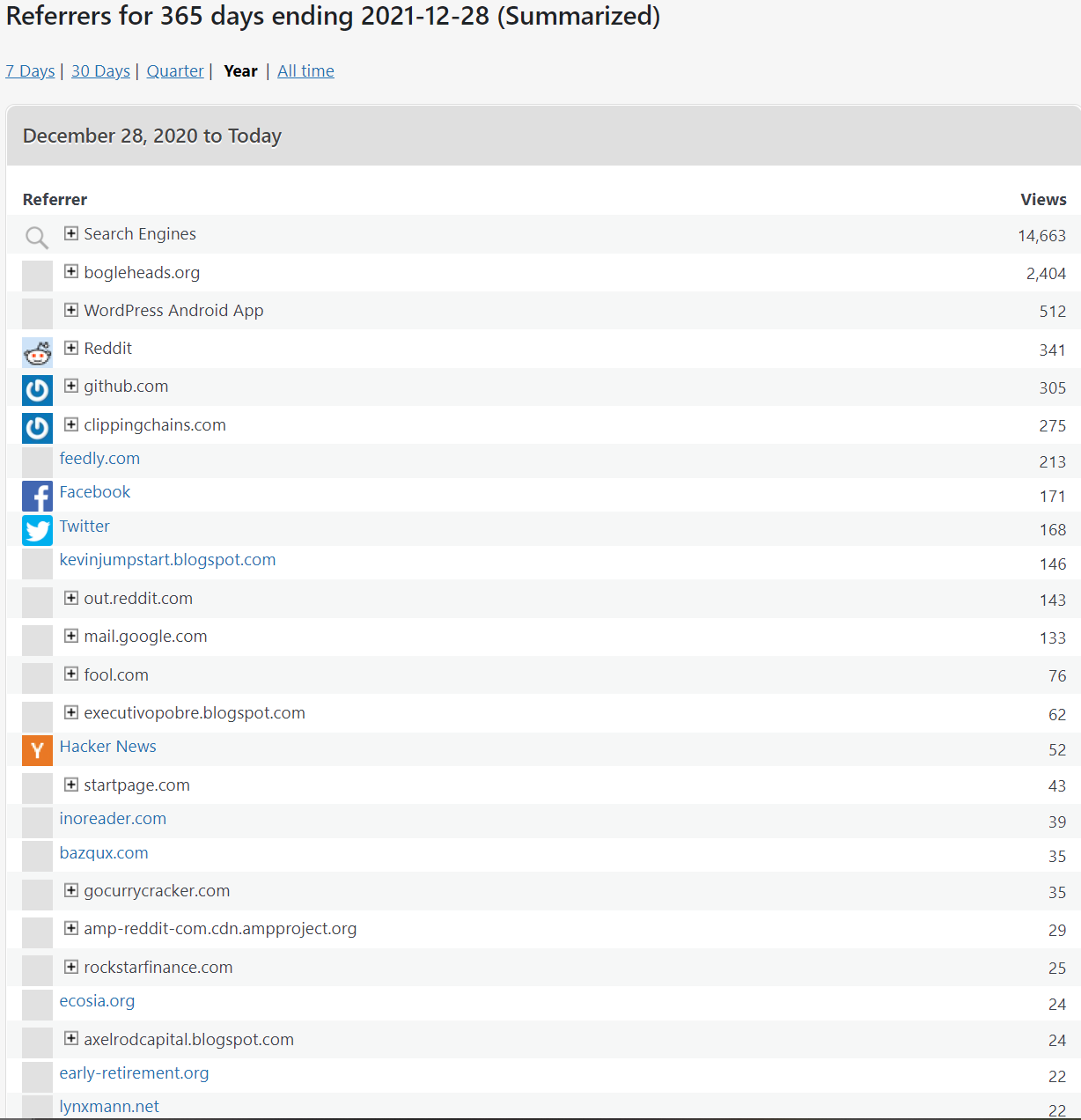The image depicts a detailed analytics dashboard with a title at the top indicating a reporting period of "365 days ending 21-12-28." To the right of the title is a summary enclosed in parentheses. Below the title, a navigation menu lists time frames: "7 days," "30 days," "Quarter," "Year," and "All time." All options are in blue and clickable, except for the "Year" tab, which is black, signifying that the current view is filtered to display yearly data.

Underneath the navigation bar, a gray header indicates "December 28th, 2022" as "Today." The dashboard is divided into columns, with "Referrer" as the title on the left column and "Views" on the right. The left column lists various referrers, some of which have expandable plus symbols for additional details. Corresponding view counts are displayed in the right column. A mix of clickable blue links and non-clickable black text represents the referrers, offering a detailed and interactive breakdown of website referrer traffic and view metrics.